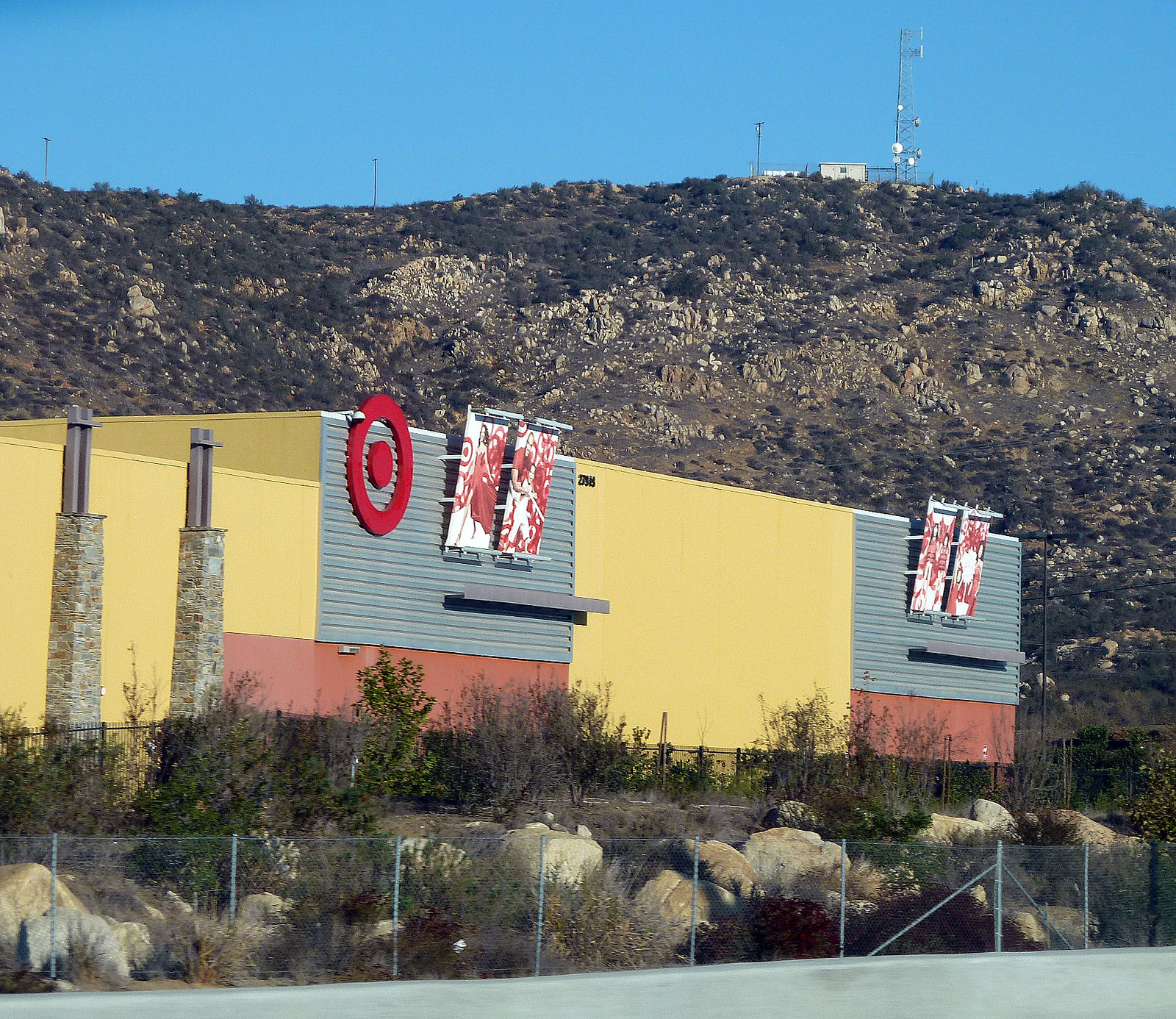The photograph captures a vibrant outdoor scene dominated by a large Target store set against a rocky hillside under a clear blue sky. The top half of the image showcases a rugged hill with scattered trees and bushes, climbing toward a metal tower connected to a small white building in the top right corner. The hillside's earthy tones contrast with the structured commercial architecture below. In the foreground, a metal fence and a rocky area lead up to the store, which features distinctive yellow walls accented by large gray panels. Prominently displayed on these gray panels is the recognizable red Target bullseye logo. The storefront is flanked by two sets of large advertisement panels on either end, with the left side also boasting chimney-like brick structures. The building's color palette transitions from the yellow walls to reddish copper and back again, giving it a dynamic, multi-hued appearance. Overall, the scene is a juxtaposition of natural ruggedness and commercial modernity.